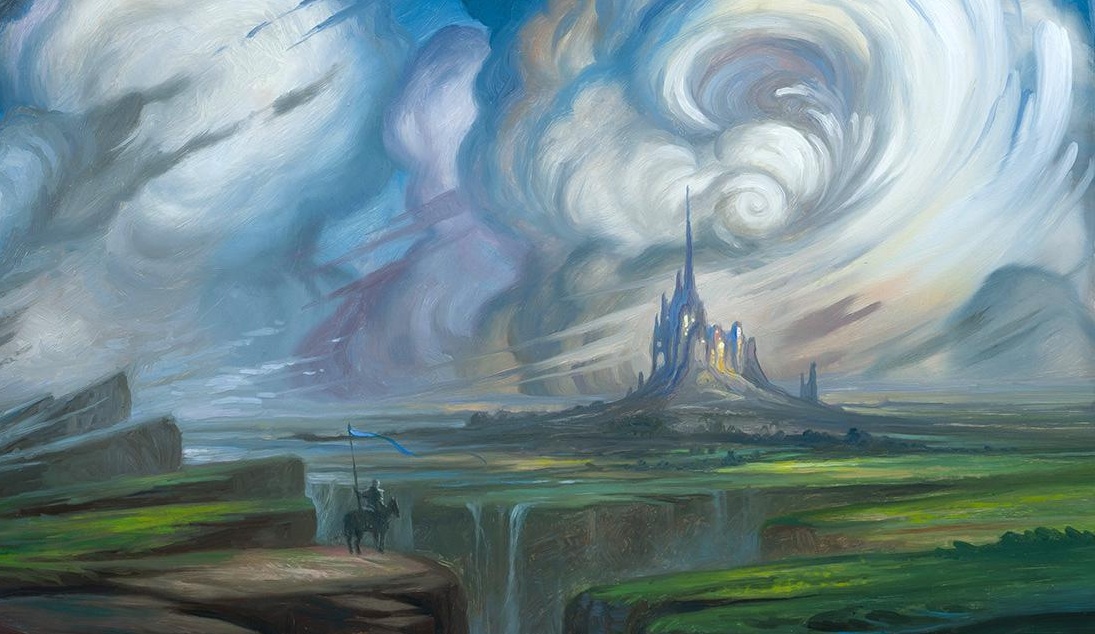The image is an intricate oil painting depicting a fantastical outdoor scene, dominated by a majestic castle. This castle, perched on a raised hill amidst a vast landscape, features four prominent spires and illuminated windows, suggesting life within. Above the castle, an enchanting sky swirls with a mix of blues, lavenders, dark grays, and whites, hinting at an impending storm.

The landscape includes a dramatic waterfall cascading in the foreground, originating from the right and contrasting beautifully with the sky. Nearby, a solitary rider on a horse stands poised on a large moss-covered rock. The rider, exuding a knight-like aura, holds a long staff with a blue flag billowing in the breeze. Surrounding them are rugged granite rocks, enhancing the wild, untamed feel of the setting. The scene's intricate details and vibrant hues combine to create a mesmerizing fantasy world, rich with narrative potential.